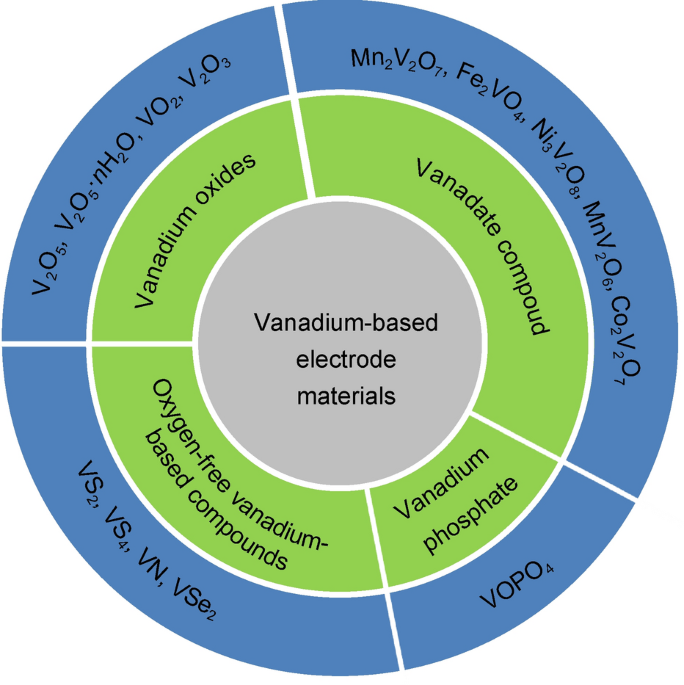The image depicts a detailed, circular, multi-layered diagram with a series of concentric rings. At the center lies a gray circle labeled "vanadium-based electrode materials." Surrounding this central circle is a green ring, segmented into four distinct quadrants, each labeled with a specific type of vanadium compound: "vanadium oxides" in the top left, "vanadium compounds" in the top right, "vanadium phosphate" in the bottom right, and "oxygen-free vanadium-based compounds" in the bottom left. Extending outward, the next layer is a blue ring, also divided into four segments. This blue ring contains various combinations of letters and numbers, such as MN2, V2, and 07, which likely represent different chemical formulas and compositions related to the vanadium compounds mentioned in the green ring. The blue segments are separated by white lines, adding a structured, segmented appearance to the outermost layer, which further emphasizes the comprehensive, reference-tool nature of the diagram. The entire layout combines to effectively convey a complex overview of vanadium-based electrode materials and their associated compounds.